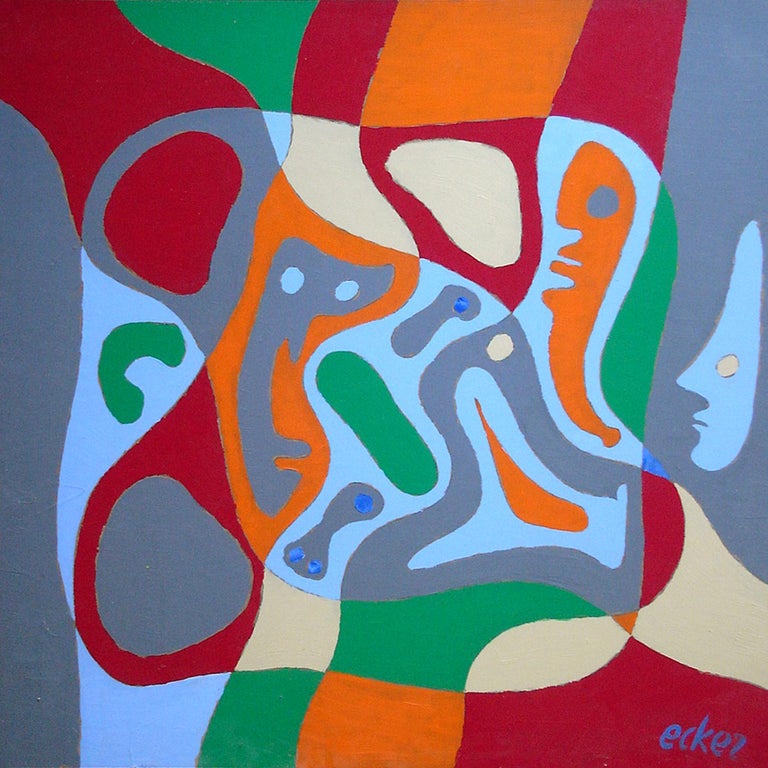This detailed, complex abstract painting predominantly features muted colors, including blue, dark gray, burgundy red, dark red, green, orange, yellow, and tan. The colors are woven throughout the composition in a way that does not make them jump off the canvas, contributing to an overall subdued effect. The painting includes various shapes and forms, such as circles, ovals, and oblong configurations, which evoke a patchwork quilt aesthetic. 

In the bottom right-hand corner, the signature "ecker," written in lowercase purple paint, is visible. Among the abstract shapes, some appear to be stylized human faces in profiles, with one notable face towards the right presenting blank eyes and a high-pointed head. Additionally, there is a gray blob with two blue spots that could suggest a cat-like form. Despite these hints of recognizable figures, the artwork remains resolutely abstract with no distinct representations of people or animals. The overall effect is a complex interplay of shapes and muted colors, creating an intricate and subtle visual experience.